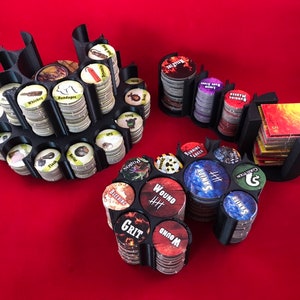The image features a vivid tableau set against a red velvet background, showcasing an array of game tokens and cards. Central to the composition is a black plastic carrel organizing various stacks of poker chips or pogs. Prominently, some of these tokens are marked with the words "wound," "grit," and possibly "warrior," in distinct colors like red, black, and blue with white text. Notably, the wound tokens are red with white check marks. Scattered across the table are diverse chips in colors including red, blue, green, and white, some adorned with caution stripes, while others feature icons like diamonds, hinting at their function as game inventory. Adding to the dynamic arrangement, there is a stack of cards to the far right and several smaller piles interspersed, all contributing to the rich, detailed scene of gaming components.